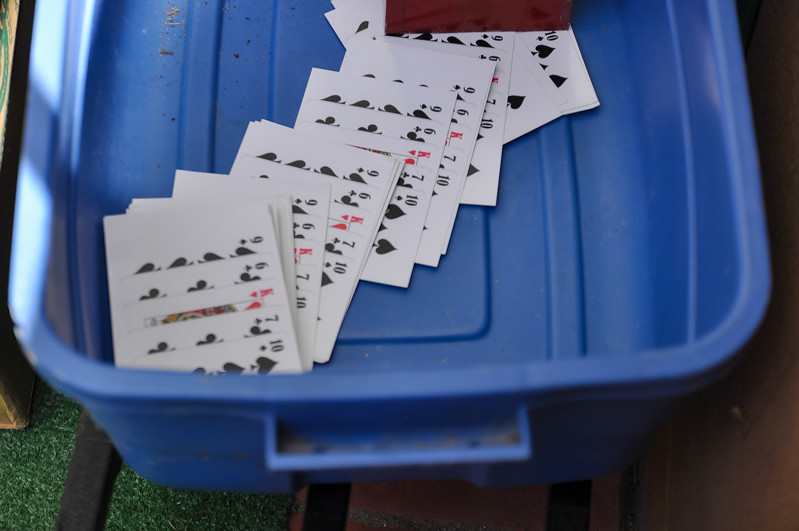This image features a large blue storage bin resembling a tub, sitting on three black bars with a layer of faux grass beneath it. Inside the bin, a variety of playing cards are scattered across its bottom, along with some visible dust and dirt. The cards are primarily from the spades suit, with multiple instances of the ten of spades, nine of spades, and six of spades. Other cards include a seven of clubs, king of hearts, six of clubs, nine of clubs, and nine of diamonds. Many of the cards are overlapping, making some of them difficult to identify. The overall scene suggests a disordered collection of playing cards primarily dominated by spades.